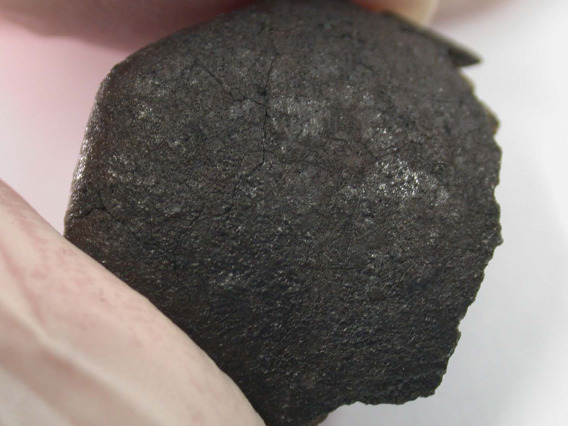This photograph is a detailed close-up of a textured, dark gray to black rock, likely a piece of charcoal or coal. The rock, characterized by its cracked and bumpy surface with bright reflections hinting at possible stickiness or wetness, is securely held between two gloved fingers. The gloves appear to be white and may be made from a protective material, underscoring the importance of safely handling this potentially dangerous specimen. The background is stark white, enhancing the focus on the rock and the gloved hands. At the very top of the image, there appears to be a squared or rectangular piece of paper or similar material placed atop the rock, possibly with another beneath it, to prevent imperfections where it is held.